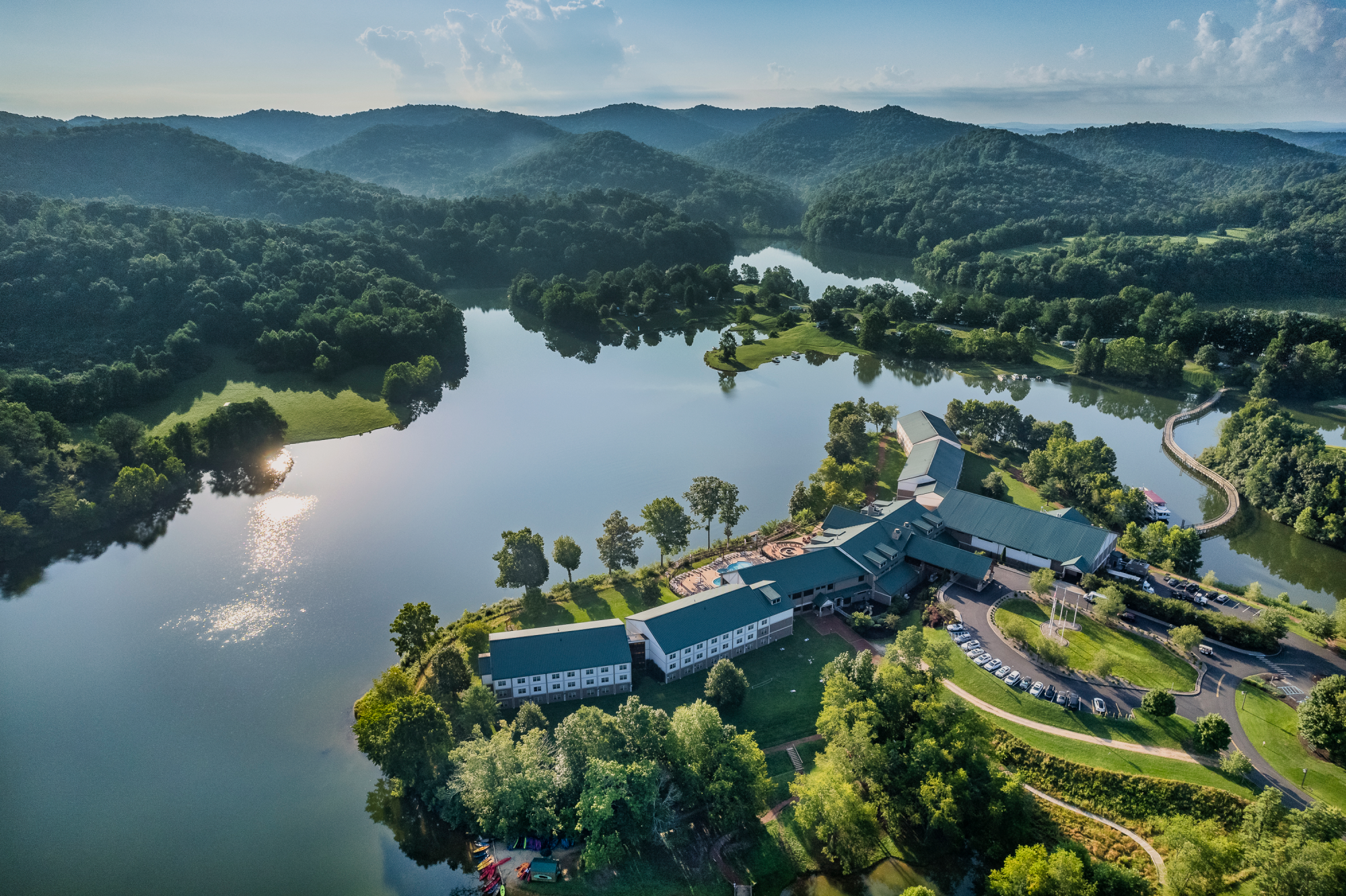This image is an aerial view showcasing a stunning landscape featuring a large lake, surrounded by a verdant expanse of green hills and mountains. The lake dominates the center of the image, reflecting the sunlight and adding a serene quality to the scene. In the distance, lush, green-covered hills and mountains rise under a blue sky dotted with gray clouds.

At the bottom right corner, a cluster of trees lines the area, interspersed with houses and buildings. A circular road, possibly a roundabout with a grassy median, is visible, with numerous cars parked along it. There is a prominent bridge that spirals across the water, enhancing the picturesque view.

Throughout the image, there are expanses of grassy fields and numerous trees, contributing to the lush greenery. Walking paths can be seen meandering through the area, indicating a well-developed landscape designed for accessibility and enjoyment of the natural surroundings. The combination of the sparkling water, the green hills, and the seamless integration of infrastructure makes this a captivating and detailed portrayal of a harmonious blend of nature and habitation.